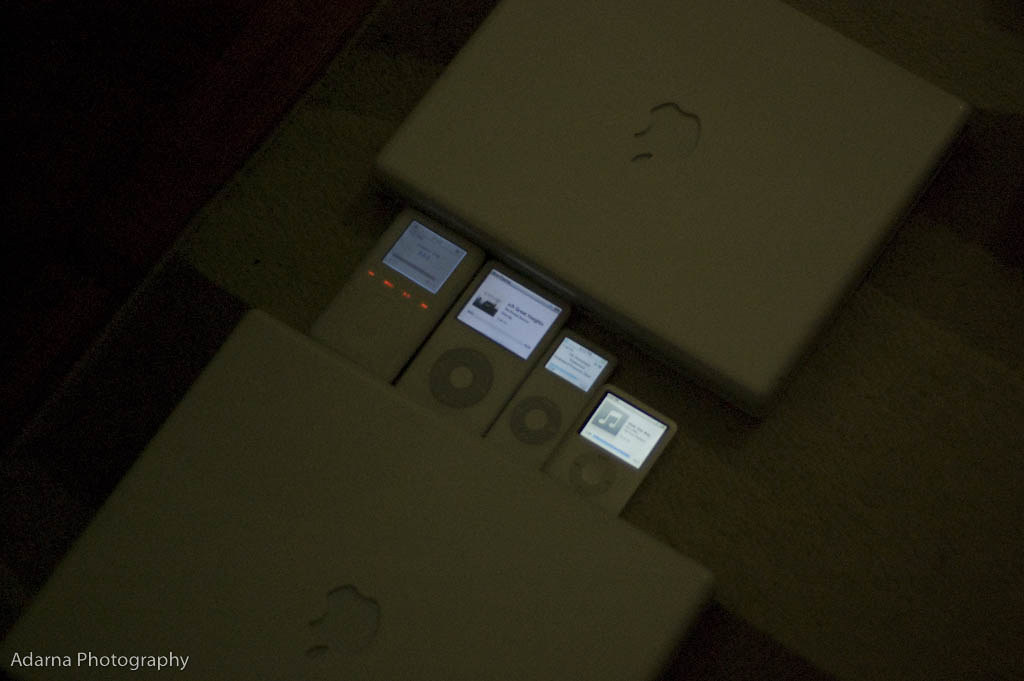This is a dark, grainy photograph with a vintage feel, credited to Adarna Photography in white text at the bottom left corner. The image prominently features four generations of iPod shuffles, arranged diagonally from the bottom left to the top right. The first iPod, larger with four faint red lights and a gray LCD screen, stands out among its smaller counterparts. Next is an iPod featuring a white LCD displaying what appears to be album art, followed by a slightly smaller, similarly styled iPod. The final iPod in the line-up is the smallest, with a screen showing a music note. All four devices rest on a desk in front of two closed, vintage iMac laptops—identified by the engraved Apple logos. The image's overall color palette is somber, dominated by dark grays, blacks, and browns, enhancing the nostalgic atmosphere.